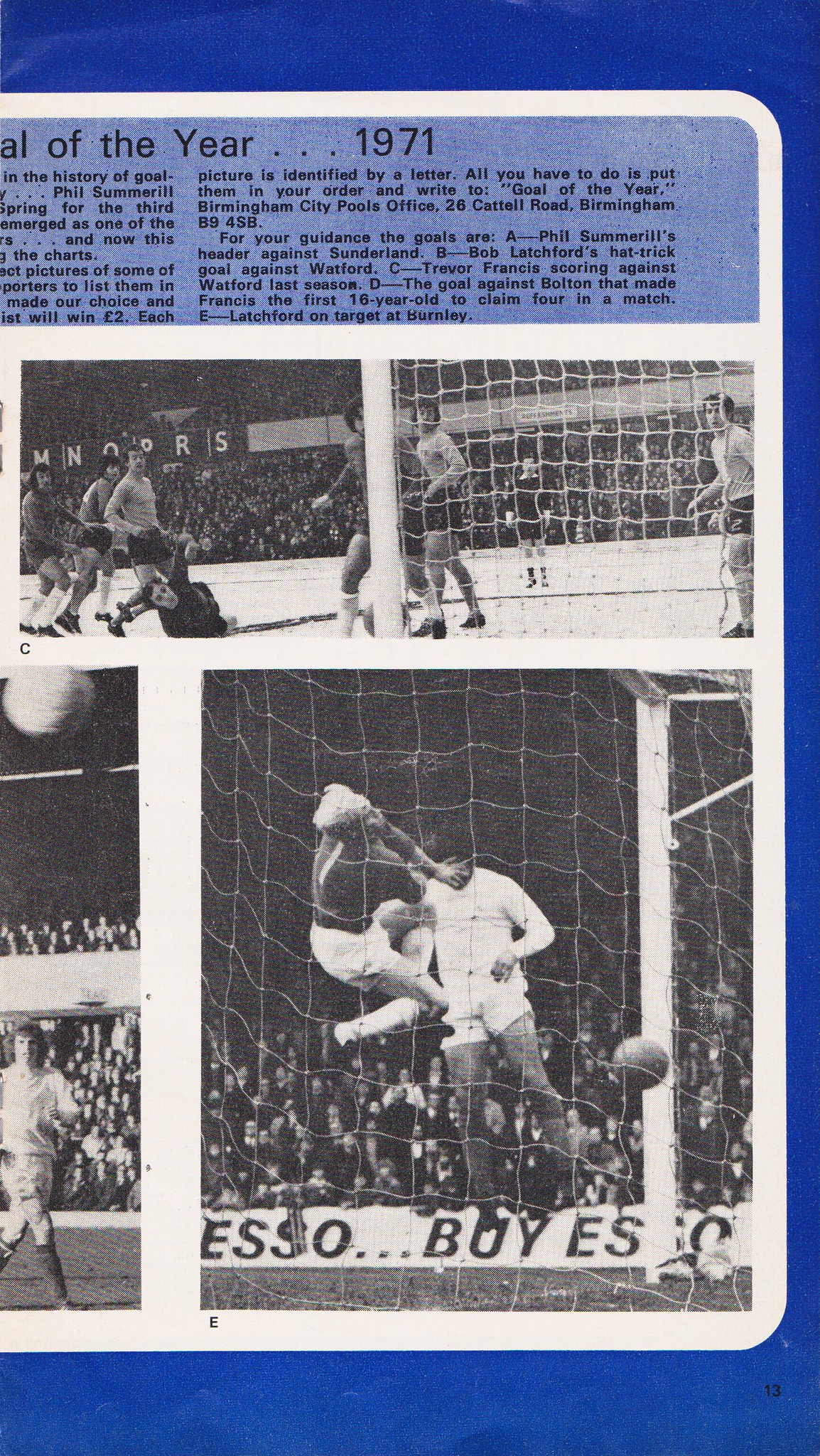This page, seemingly from a 1971 European football magazine, prominently framed in a royal blue border, features a black-and-white collage of iconic soccer moments. Labelled images, arranged in a grid formation, capture historic goals and their scorers. The top paragraph details the significance of each image: A showcases Phil Summerill's header against Sunderland; B features Bob Latchford's hat-trick goal against Watford; C portrays Trevor Francis scoring against Watford from last season; D highlights the historic goal making Francis the first 16-year-old to score four goals in a single match against Bolton; and E depicts Latchford on target at Burnley. Notably, photo C appears as a split image due to the goalpost divider but is part of a single picture sequence. The provided text, aimed to engage the readers, invites them to match the images to their respective descriptions and submit entries for a 'Goal of the Year' competition via the Birmingham City Pools Office.